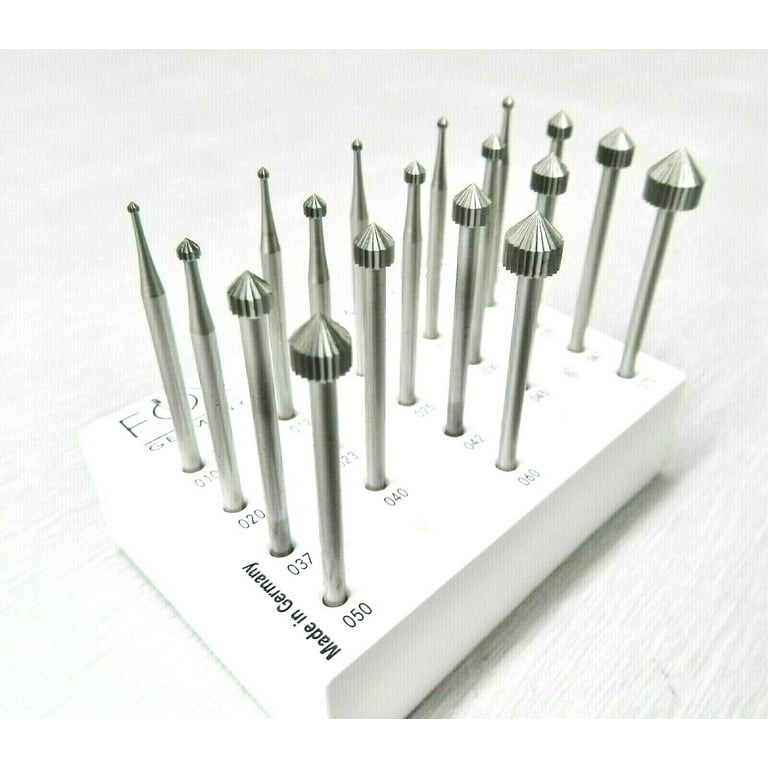The image features a small white tray, likely made of plastic or metal, sitting on a white wood grain surface, photographed at a diagonal angle. The tray is a 3D rectangular shape and bears the text "Made in Germany" in the bottom left-hand corner. Additionally, there is partially visible text at the top reading "F.O. Germany." The tray is perforated with numbered holes, from which various metal pegs protrude. These pegs, about 18 in total, appear to be drill bits or control pins of equal length but with differently sized, pointed heads that feature flanges and ridges. Each peg is labeled with numbers, such as 50, 37, 20, etc., indicating either their size or model numbers. The front row of holes is numbered sequentially from 1 to 50, while the second row ranges from 12 to 40, emphasizing a meticulous organizational system.